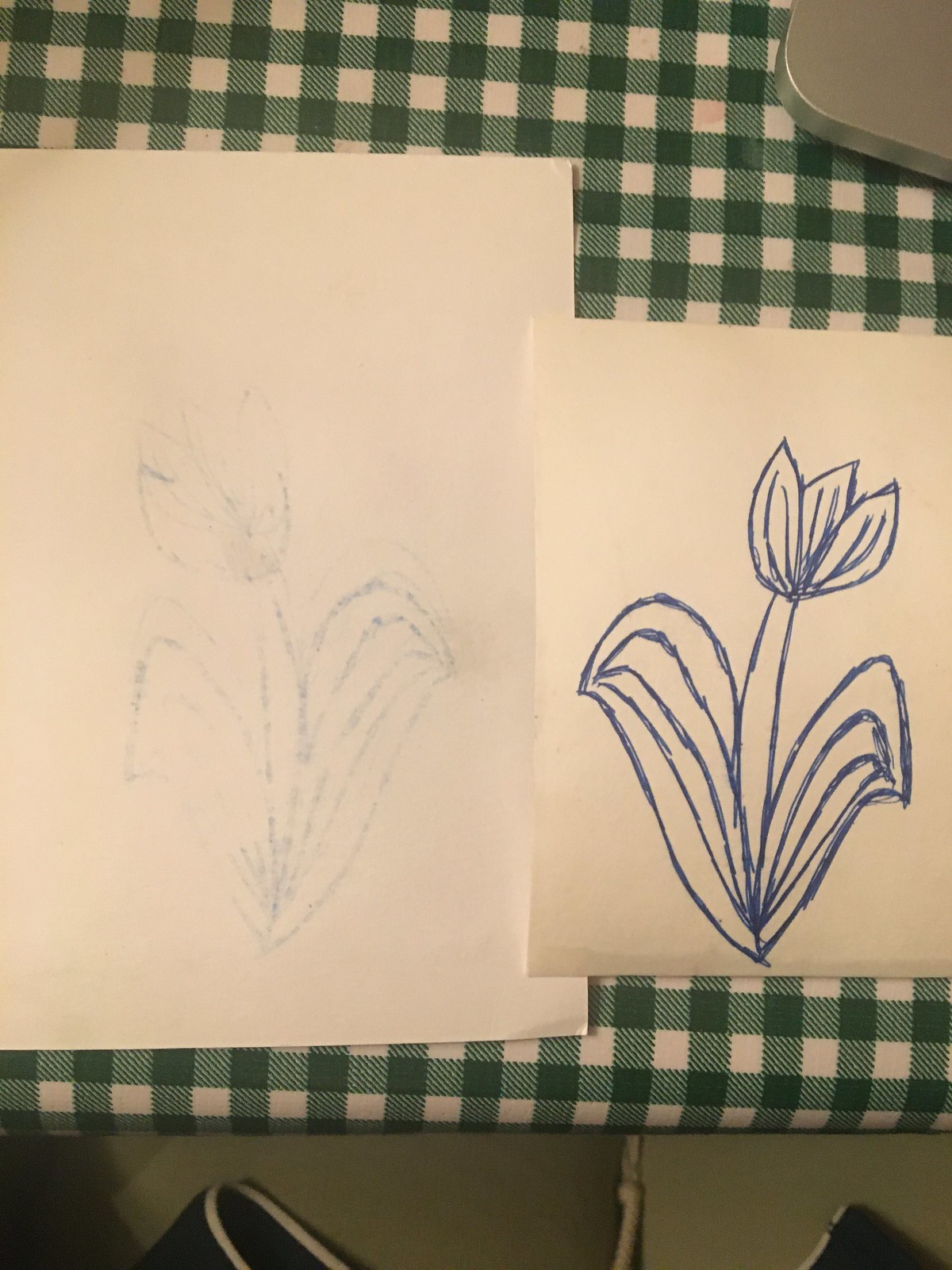The image captures a detailed scene of artwork setup on a table. The table is draped with a green and white checkered tablecloth, underneath which a hint of gray, possibly the table's surface, is visible. At the bottom of the image, the heels of two shoes can be seen, adding a subtle human element to the scene. The focal point consists of two sheets of white paper. The larger sheet on the left shows a faint imprint of ink, suggesting it was used to blot excess ink from the smaller sheet on the right. The smaller, overlapping sheet features a bold, blue ink drawing of a tulip, complete with three petals, a stem, and two leaves. The blue ink lines are thick, indicating that they were traced over multiple times. In the upper right corner of the photograph, part of a rounded metal pencil case peeks into the frame. The overall setting is casual, likely atop a picnic table given the context.